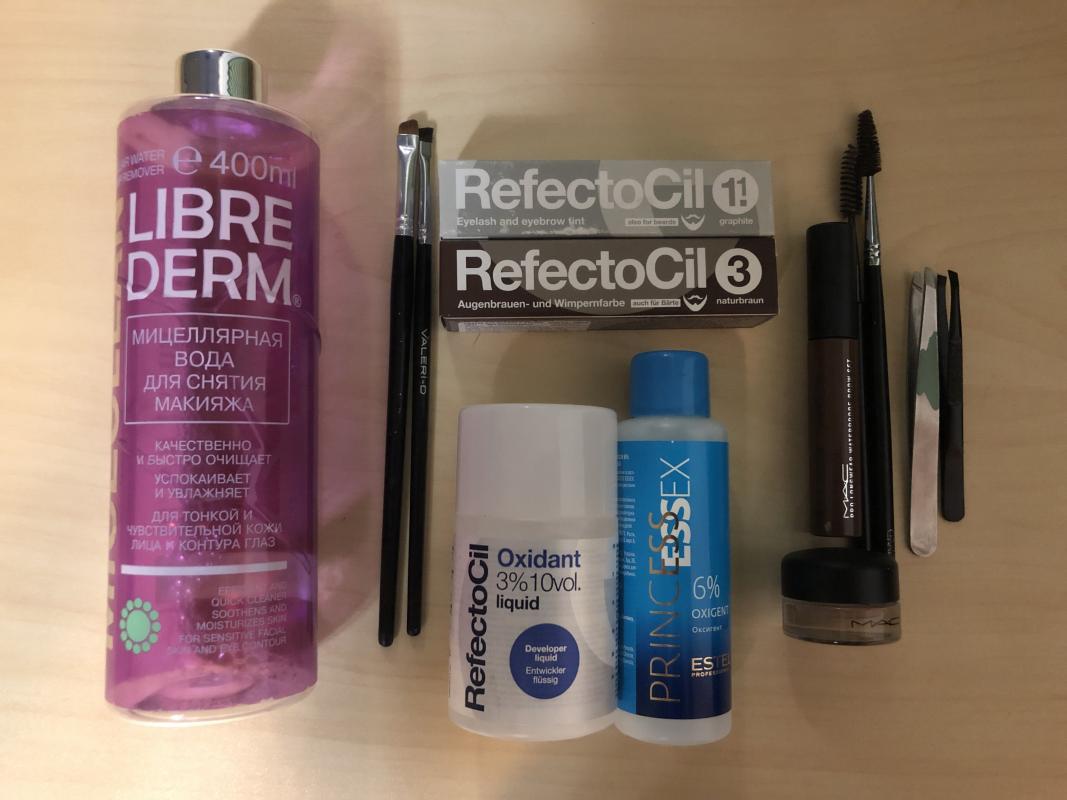Top-down photograph of an assortment of beauty products meticulously arranged on a cream-colored wooden table. The light source on the left creates a stark contrast with the shadow cast on the right, presumably from the person taking the photo.

The items are organized vertically from left to right:
1. A large, pinkish-purple bottle branded "LibraDerm," featuring Cyrillic text, suggesting it may be a Russian product, though the specific type of product remains unclear. The description reads "car water remover."
2. To the right of the bottle, two small brushes with black handles and a small silver-aluminum coating. The bristles are short and brown.
3. Directly to the right of the brushes, two packages labeled "RefectoCil" are positioned at the top. 
4. Below the "RefectoCil" packages is a white bottle labeled "RefectoCil Oxidant Liquid."
5. Next to the white bottle is a blue bottle labeled "Princess Essex." 
6. To the right, a small bottle branded "Mac" is visible.
7. Above the "Mac" bottle sits a brown bottle, and to the right of this are several applicators.
8. Completing the arrangement, two pairs of tweezers are placed adjacent to the applicators.

This arrangement showcases a variety of beauty products and tools, offering a visually pleasing and organized display.